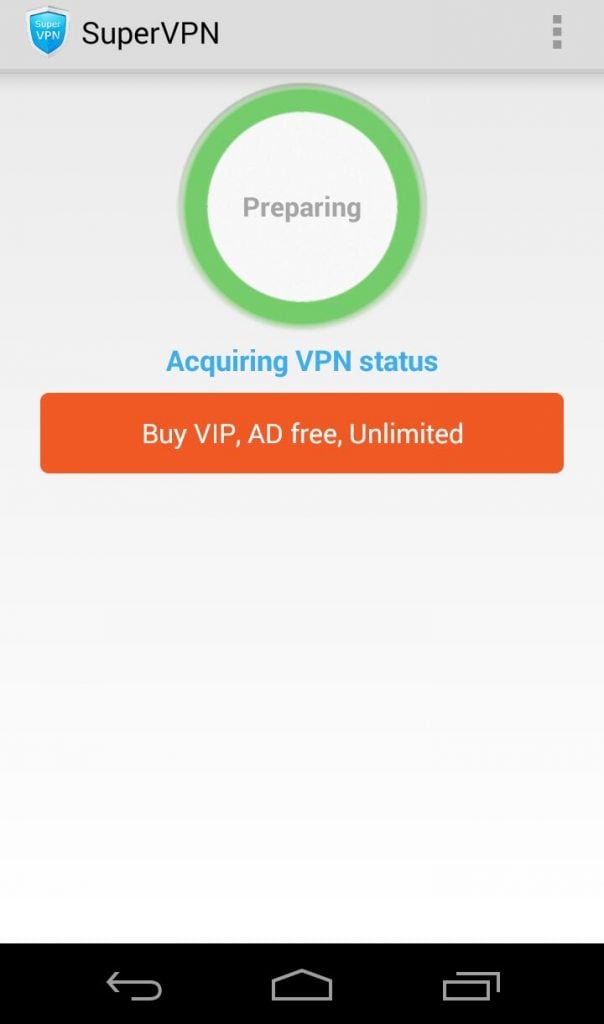The image displays a smartphone screen showcasing the SuperVPN application. At the bottom of the screen, the familiar smartphone navigation icons are visible, including the back button, home page button, and the app minimization button (depicted as a double box).

At the top, within the application's header, there is a blue badge labeled "SuperVPN" with specific capitalization: "S" in "Super" and "VPN" entirely in uppercase. Adjacent to the badge on the right side are three vertical dots, presumably indicating a menu or additional options.

The main section of the app displays a status labeled "Preparing" within a central circle, which is highlighted by a green progress bar encircling it. Below this, the text "Inquiring VPN status" appears in blue.

Further down, there is a prominent red box containing the text "Buy VPN, ad-free, and unlimited," indicating a premium purchase option for enhanced features.

The background of the app is a very light gray, almost white, providing a clean and uncluttered interface.

Overall, the caption details that the application shows the VPN status as "preparing," provides an option to inquire about the VPN status, and offers a purchasable upgrade for ad-free and unlimited access.